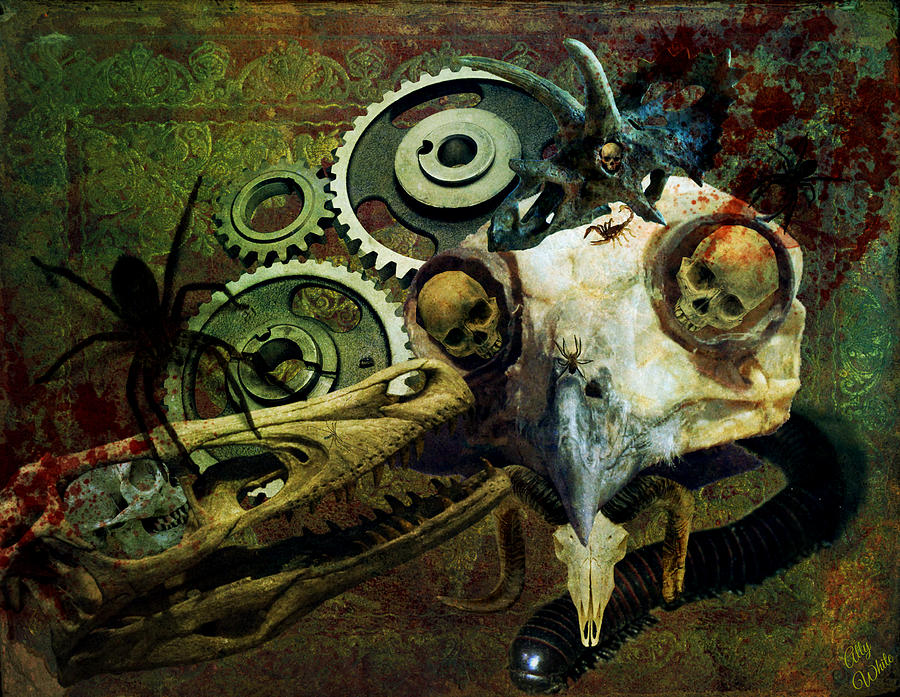The artwork is an intricate and darkly abstract illustration characterized by a haunting array of elements. Dominating the scene are two prominent human skulls situated centrally and to the right, surrounded by creepy crawlies—most notably, a large black spider and a smaller one, allied with a menacing scorpion. Not merely confined to the macabre, the painting integrates mechanical aspects, including several metallic gears, prominently positioned in the upper left corner, with a black spider perched on them. A striking feature is an animal skull, likely from a goat or ram, situated in the bottom middle, with a dramatic hawk or bird skull in the center right, notably harboring two human skulls within its eye sockets. Below this avian structure slithers a large centipede, while above lurks a more cryptic dinosaur skull, possibly a velociraptor or triceratops, again housing a human skull within its recesses. These elements are tied together in a collage-like manner, with the stark contrast of dark colors providing a chilling coherence. Additionally, the artist's signature, "Ali White," discreetly adorns the bottom right of the composition, beneath a centipede, adding a personal mark to this eerie tableau.